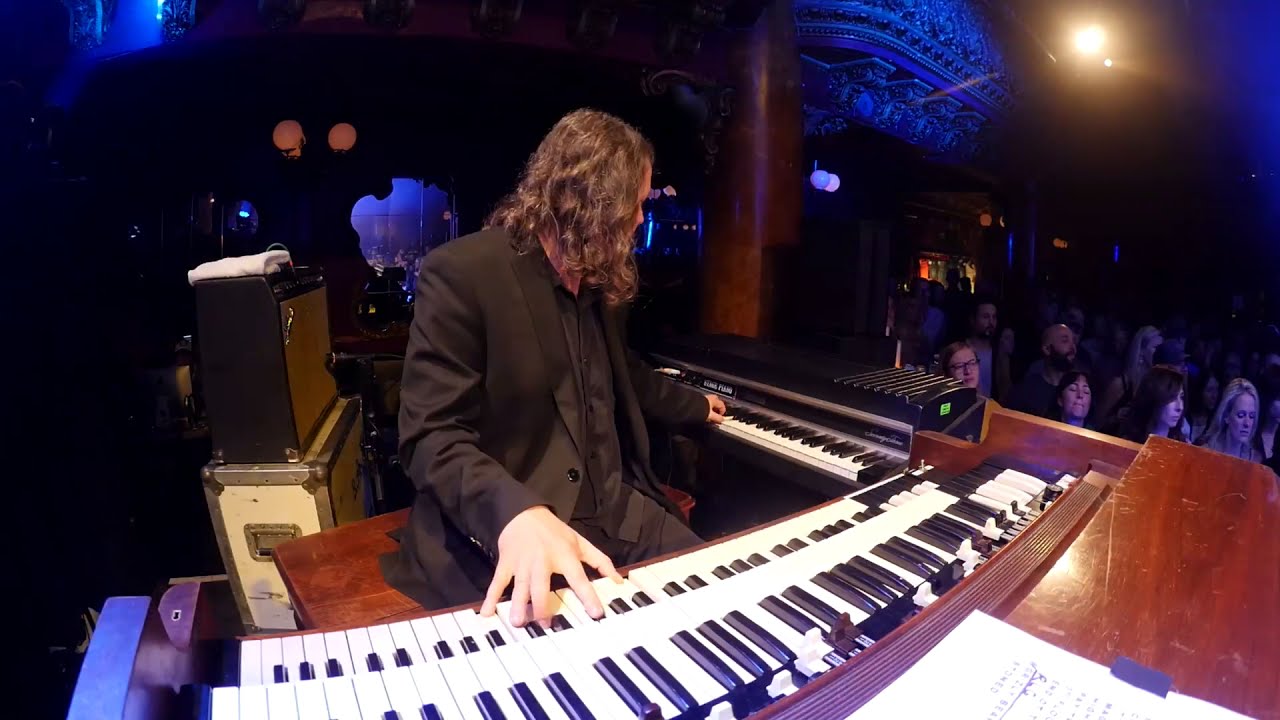The photograph captures a live performance by a Caucasian male keyboardist with shoulder-length, slightly wavy brown hair, which is pushed back from his forehead. Clad in an elegant black suit and black shirt, he commands attention at his illuminated station on stage. Positioned in an L-shaped arrangement, he skillfully plays two sets of keyboards simultaneously, each with one hand—his left hand over a synthesizer and his right over another keyboard with a distinctive wooden top. The stage setup also includes a setlist on the wooden desk beside him. The scene is set in a nightclub or bar, with dark surroundings punctuated by blue lights and spotlights. Behind him, equipment and possibly a mirrored wall reflecting the bar can be seen. The audience, primarily composed of women, flanks the right side of the frame, watching intently. The image background consists mostly of the dimly lit stage area, emphasizing the lively yet intimate atmosphere of the indoor venue.